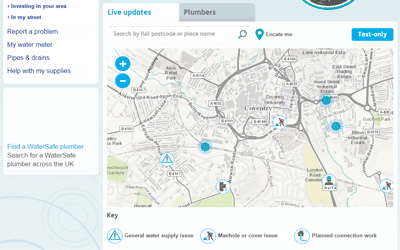Caption: 

The image depicts a detailed website interface centered around a map, aimed at assisting users with various water-related services. On the left sidebar, several options are listed including "Invest in Your Area," "Report a Problem," "My Water Meter," "Frozen Pipes and Drains," "Help with My Supplies," and "Find a Winter Sale Plumber." A search field allows for locating a water sale plumber across the UK, emphasized in blue text. 

The main content area prominently features a map, rendered in shades of brown, tan, and cream, punctuated by two blue circles indicating zoom in (+) and zoom out (-) controls. A banner in blue reading "Live Updates" is displayed at the top. 

Above the map, there's a search browser labeled "Plumbers," and to the right, a light teal sidebar partially reveals a teal circle with a brown inside. The map itself is designed with a mix of blue and white spots, each containing small images, indicating different features or locations. A small blue box marked "Test Only" is visible on the map. Below the map, three sections are presented, each accompanied by images and descriptive text. The word "Key" is positioned at the top of this segment, helping users to decode the map symbols and colors.